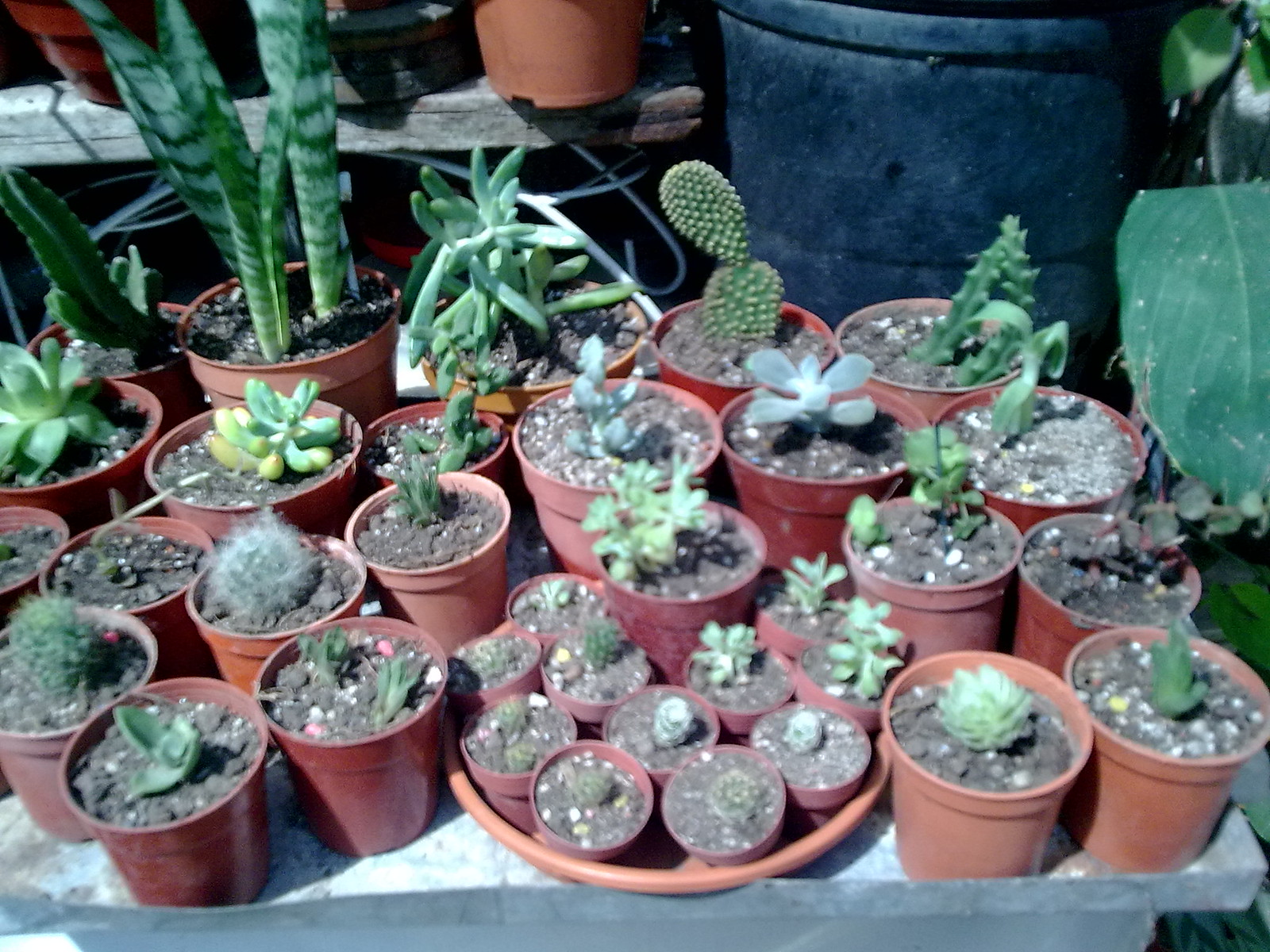The image showcases a diverse collection of approximately 20 to 25 potted plants, predominantly succulents and cactuses, positioned on an outdoor table. The plants are housed in light and reddish-brown terracotta-like plastic pots of various sizes, with many of the small pots gathered in a circular tray, which appears to be the saucer of a larger terracotta pot. The soil in the pots looks quite dry, suggesting the plants have not been watered recently. Among the variety, one can observe not only cactuses but also some tropical plants, including a tubular green plant, a green cactus, a jagged-edged green plant, and a slightly purple plant. Taller green and white stems are found on the left side. Dominating the top right of the scene is a large bluish pot with a noticeably large green leaf beside it. The backdrop features a significant black barrel and additional larger plants in pots, contributing to the tableau of an outdoor garden space in need of a bit of care.